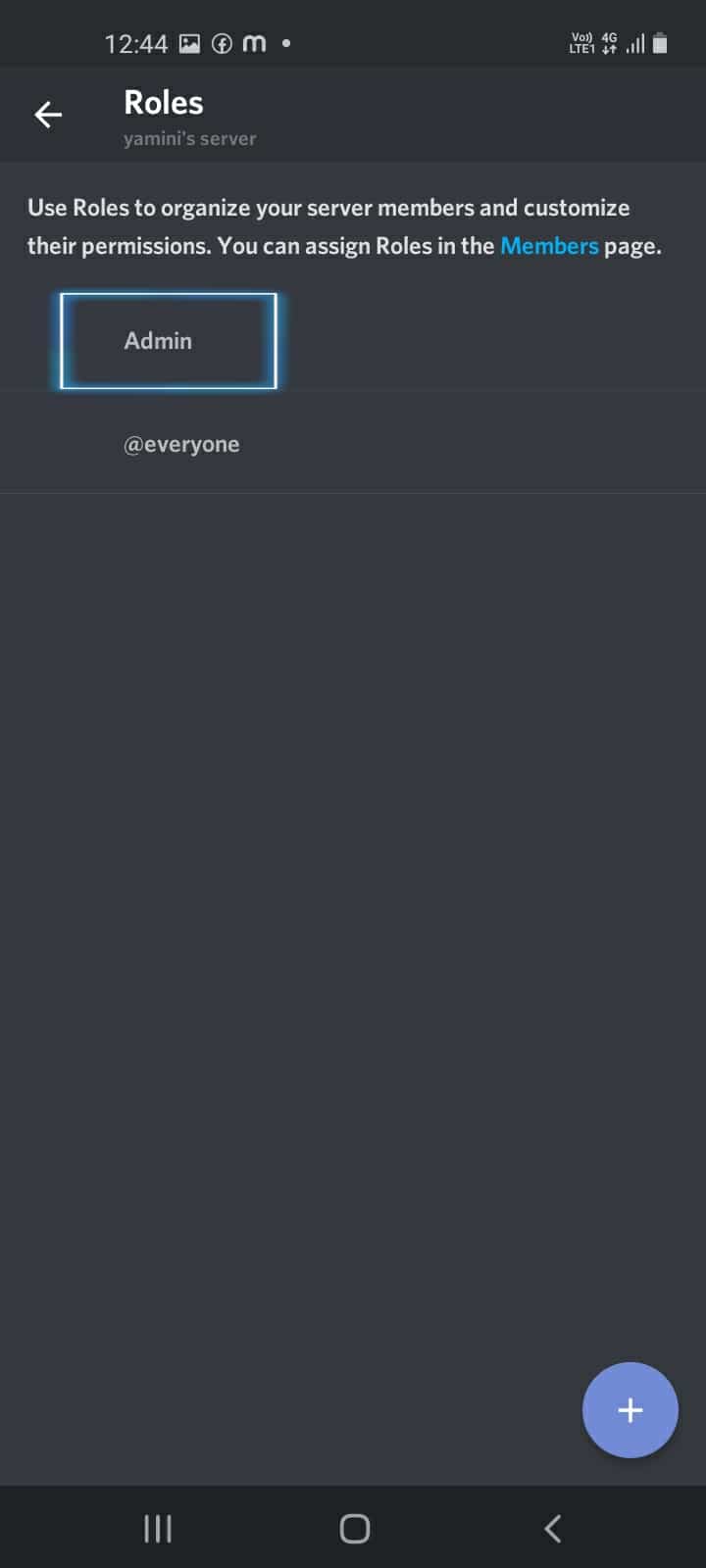The image is a tall rectangle, approximately twice as tall as it is wide, with a dark gray to black background.

At the very top, there is a black bar containing several white elements: the number "1244" at the leftmost side, followed by a picture icon, an information icon, and a small letter "M". On the right side of this bar, there are multiple icons indicating battery status and charge level.

Below this top bar, in very dark gray with white text, the word "Roles" is prominently displayed. To the left of "Roles," a white arrow points to the left. Directly underneath "Roles," in smaller, light gray lowercase letters, is the text "Yamini's Server."

Further down, the background lightens slightly but remains dark gray. In white letters at the top of this section, the text reads: "Use Roles to Organize Your Server Members and Customize." On the line directly below, it continues: "Their Permissions." This sentence is followed by a period. The word "Members" within this text is highlighted in Tiffany Blue and has a capitalized 'M'.

Directly beneath this messaging, there is a blue and white rectangle. Centered within this rectangle, on the dark gray background, the word "Admin" appears in light gray letters. Below this, still on the dark gray background, the word "@Everyone" is displayed in light gray lettering. Here, the "@" symbol is stylized with the 'A' inside a circle.

At the very bottom of the image, there is a black band featuring three vertical lines on the left, a square with rounded edges in the middle, and an arrow pointing left on the right. Just above this black band, located at the bottom right of the dark gray section, there is a medium-large light purple circle containing a white plus sign.

This image seems to be a user interface screen possibly from a server management or communication application.